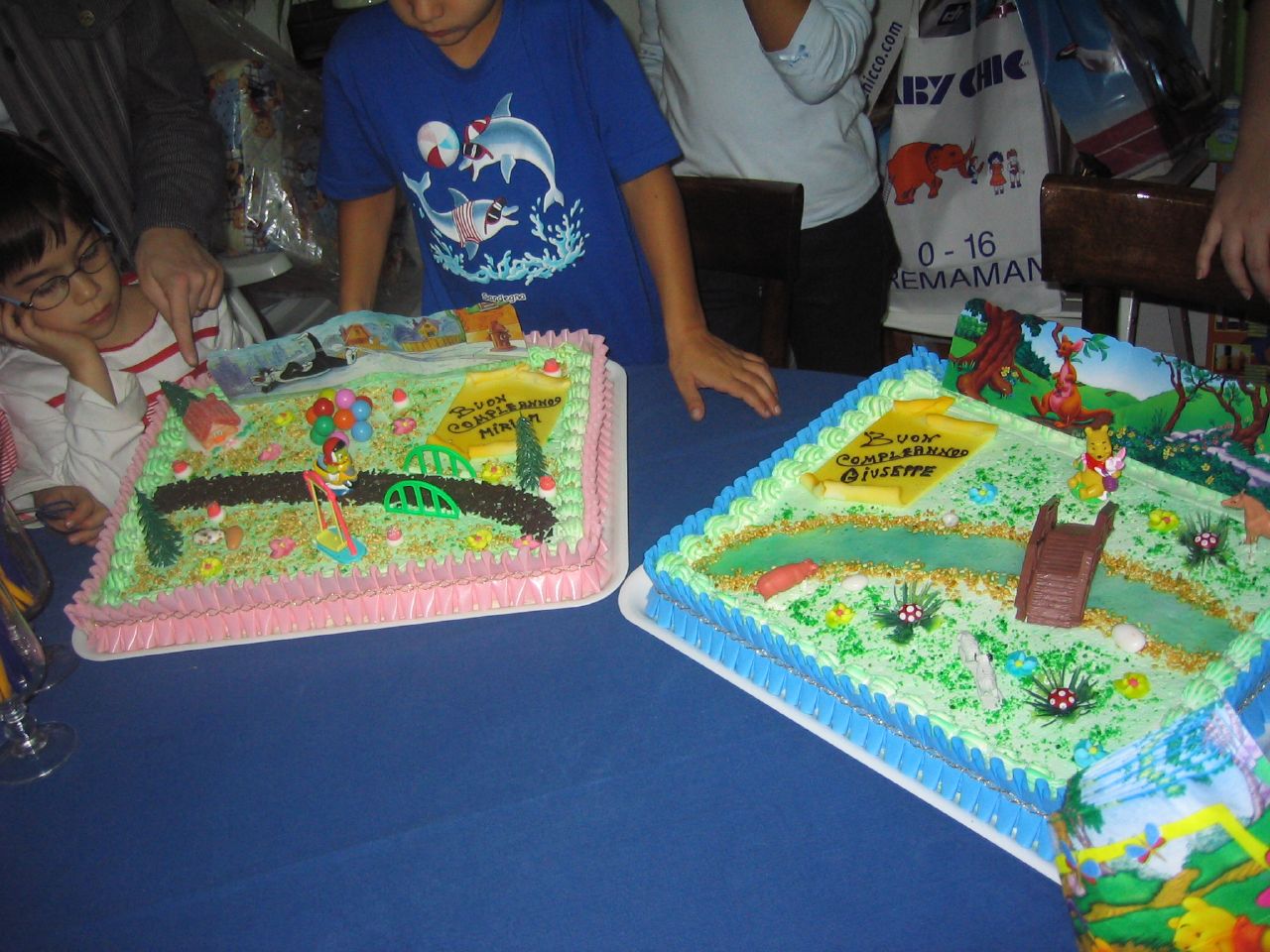The image captures an amateur photograph of a children's birthday party, slightly dark, showcasing two elaborately decorated birthday cakes on a large, circular table covered with a blue tablecloth. Both cakes, designed in equal size and rectangular in shape, seem to cater to a boy and a girl, as indicated by the color themes—pink for the girl and blue for the boy.

The cake on the left is pink, featuring intricate frosting designs that depict an outdoor scene: a green path resembling a bridge, colorful egg-shaped decorations, a small frosting house, several trees, and a play swing. The cake is inscribed with "Buon Compleanno Miriam" on a frosting scroll, partially obscured by a tree, along with a cute penguin holding balloons.

The cake on the right is blue and carries a woodland theme with a river, a brown bridge, and green grass. This cake is adorned with Winnie the Pooh and Piglet figurines, mushrooms, and has the message "Buon Compleanno Giuseppe" in black text on an orange frosting scroll.

In the background, children are visible, seemingly less excited but observant. On the left, a little girl with her head resting on one hand is shown having an adult's hand over her shoulder, pointing at the little house on the pink cake. Beside her is a boy in a blue shirt with dolphins printed on it, focused on the pink cake. Around them are adults, including one in a white shirt and black pants, holding a bag that says "Baby Sheik," and another resting a hand on a brown chair. 

The overall ambiance suggests a joyful twin or siblings' birthday celebration, highlighting the joy and creativity poured into the cakes' designs and the shared moment among the children and adults present.